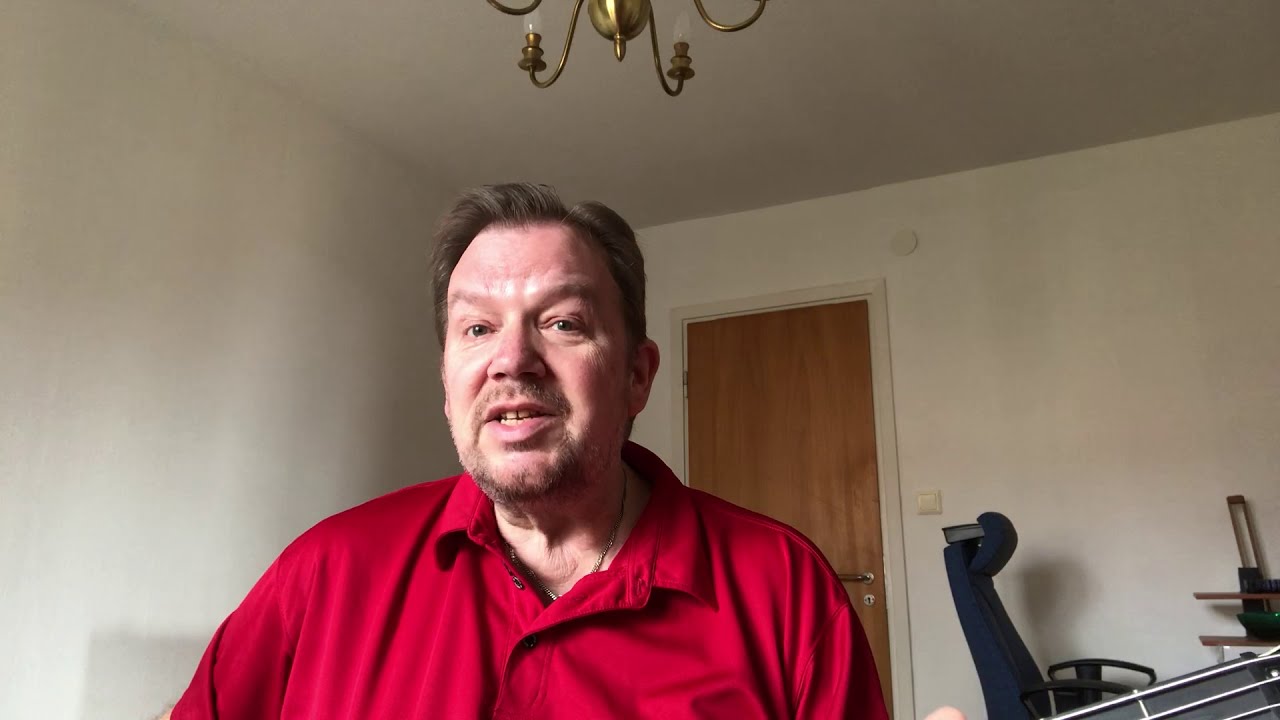This is a photograph of a middle-aged Caucasian man with short brown hair, a slight gap between his front teeth, and visible facial hair, including a light-colored mustache and goatee. He is wearing a red polo-style collared shirt, buttoned down the front, with a pocket on the left side that might have a logo or writing on it. The shirt has a slightly open collar, and he is also wearing what appears to be a silver chain around his neck. The man is pictured from mid-chest up, facing directly into the camera with his mouth slightly open as if he might be speaking.

He is inside a room with white walls and ceiling, lit by natural light coming from a window, which falls on his face. Behind him, over his left shoulder, is a closed wooden door. Directly above his head, you can see part of a gold-colored light fixture, possibly a candelabra-style chandelier with multiple arms, though it is turned off. To his right, the background includes a navy blue office chair and a desk, and a pile of indistinct items partly visible in the bottom right corner of the image. The overall setting suggests an interior space, possibly a living or dining room within a house.